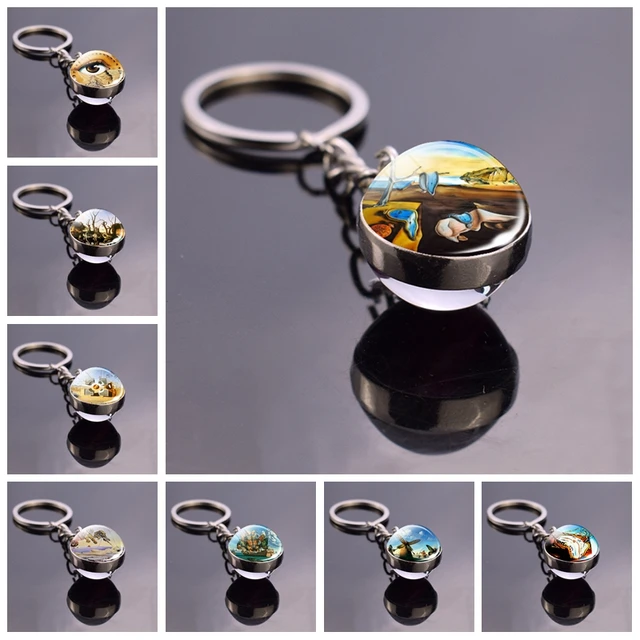The image is a collage showcasing various keychain designs on a gray background. The main focus is a large square on the top right, depicting a close-up of a keychain with a decorative marble. The marble features the famous Salvador Dalí painting "The Persistence of Memory," known for its melting clocks. The keychain's silver ring is positioned in the upper left, connected to the marble via a silver band and a small chain. A subtle drop shadow is cast below the keychain.

Down the left side of the image and extending across the bottom, there are eight smaller squares displaying different keychain designs, each with a unique decorative marble. The designs include an eyeball, a forest scene, various outdoor landscapes, a ship, a windmill, and another depiction of a melting clock. The reflective surface beneath the keychain in the central image adds a black mirrored reflection, enhancing the overall visual appeal.